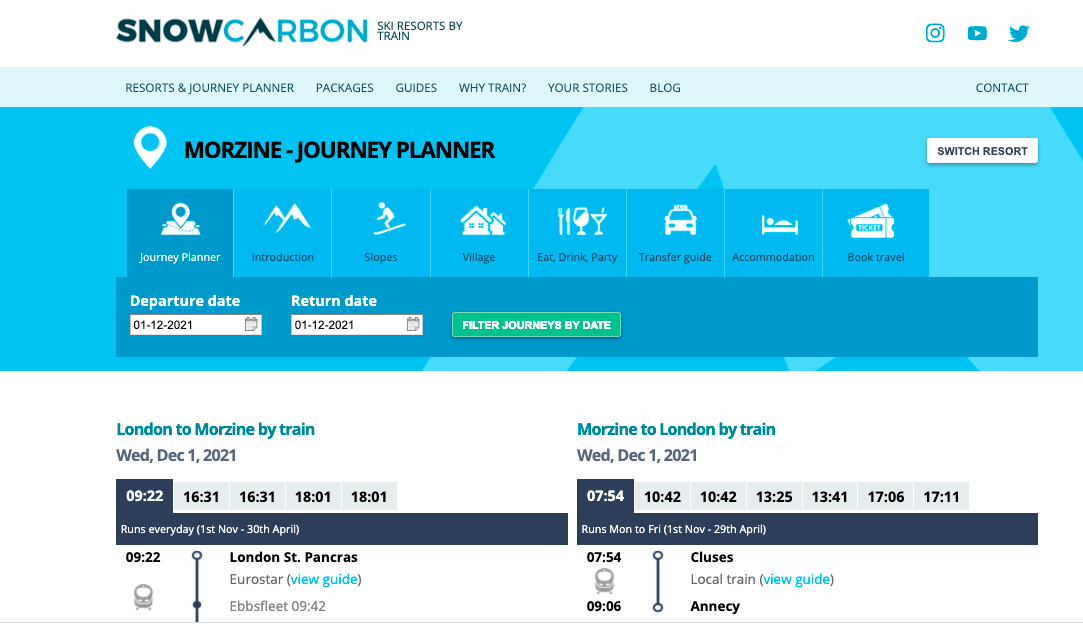In this image of the Snow Carbon website, the design is visually striking and meticulously organized. The logo features the text "carbon" with a unique 'A' that resembles a mountain, evoking a sense of adventure. Prominently displayed, the header includes icons for Instagram, YouTube, and Twitter on the top right, facilitating easy access to social media channels.

Directly below, a blue banner background hosts a lighter blue tab with navigation options including "Resorts and Journey Planner," "Packages," "Guides," "Why Train," "Your Stories," "Blogs," and "Contact" on the far right. Beneath this, a darker blue section catches the eye with a location emoji and the label "Morzine Journey Planner" in black letters. To the right of this, there's a clickable "Switch Resort" button with a black rectangle background.

Further down, a variety of planning tools are available: an icon for the Journey Planner is followed by sections for "Introduction," "Slopes," "Village," "Eat," "Party," "Drink," "Transfer Guide," "Accommodations," and "Book Travels." Users can select their departure and return dates via a mini calendar feature. Finally, a prominently placed green rectangular bar labeled "Filter Journeys by Date" allows users to refine their travel plans efficiently.